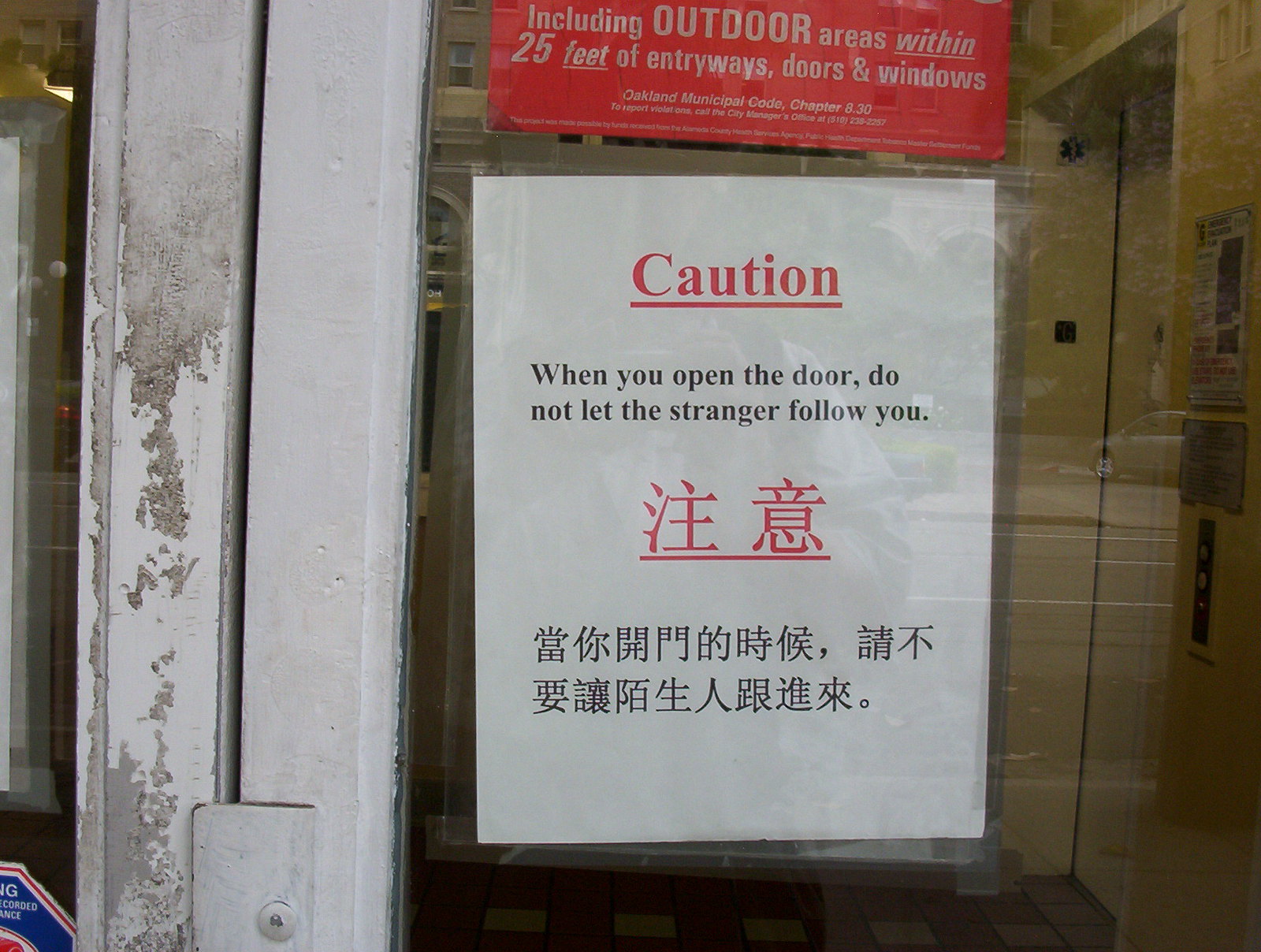The image depicts an old glass door with a white metal frame, showing signs of wear and peeling paint. Two signs are taped to the door. The top sign is red with white text, which reads, "Including outdoor areas within 25 feet of entryways, doors, and windows. Oakland Municipal Code, Chapter 830." Below it, a white sign with red and black text warns, "Caution: When you open the door, do not let the stranger follow you." Additional text on this sign is written in either Japanese or Korean. Through the glass, on the right side of the frame, an elevator is visible, suggesting the door likely leads to an apartment complex or a similar multi-story building. No people are present in the scene.